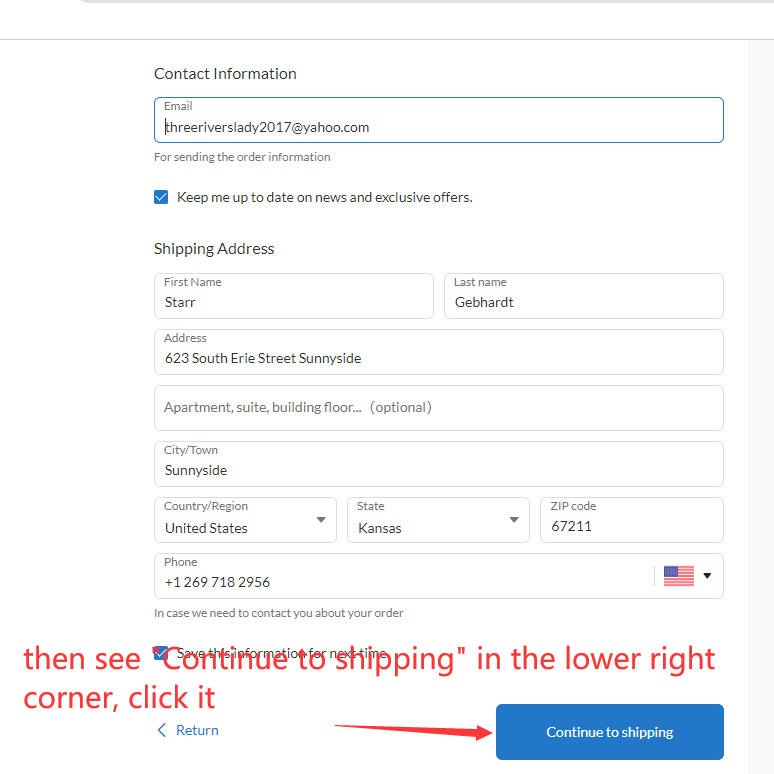The form is meticulously structured for entering contact and shipping information:

1. **Contact Information Section:**   
   - At the top and bottom of the section are horizontal grey divider lines.
   - Between these lines is white space followed by bold, black text stating "Contact Information".
   - Below this header is a blue rectangle bordered in white, containing fields to enter details.  
     - It prompts for an email address and displays an example entry as "3RiversLady2017@yahoo.com."
     - There is a checkbox, blue with a white checkmark, labeled "Keep me up to date on news and exclusive offers".

2. **Shipping Address Section:**  
   - There is a header reading "Shipping Address" followed by multiple fields framed with grey borders.
   - The form includes fields for:
     - **First Name:** Entered as "Starwick" (with a note of "2Rs" indicating double 'R').
     - **Last Name:** Entered as "Gebhardt" (noted as G-E-B-H-A-R-D-T).
     - **Address:** Entered as "621 South Erie Street, Sunnyside".
     - **Apartment, Suite, Building, Floor:** This is optional and left blank.
     - **City/Town:** Entered as "Sunnyside".
     - **Country/Region:** Selected as "United States".
     - **State:** Selected as "Kansas".
     - **ZIP Code:** Entered as "67211".
     - **Phone Number:** Entered as "+12677182956".
   - Following the phone number field, there is an American flag icon with supplementary text: "In case we need to contact you about your order".

3. **Continue to Shipping:**  
   - At the bottom right corner, there is a red arrow pointing towards a blue box that says "Continue to Shipping" in white text.